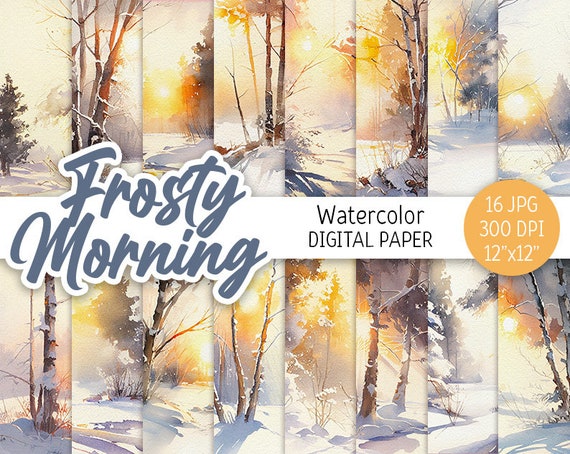The image is a cover for watercolor digital paper titled "Frosty Morning," displaying a collection of 16 wintry scenes in landscape mode. At the top, "Frosty Morning" is written in dark blue cursive, centered between two orange circles that read "16 JPG, 300 DPI, 12x12 inch." Each scene features different angles of leafless trees and snow-covered ground, with a creamy-colored sky illuminating the landscape. The images capture the sunrise casting long, gray shadows on the snow, highlighting the intricate details of pine trees, birch-like trunks, and occasional golden leaves bathed in sunlight. The consistent theme of a cold, frosty morning is evident as the sun rises behind the trees in each frame, creating a serene and detailed portrayal of a winter landscape.